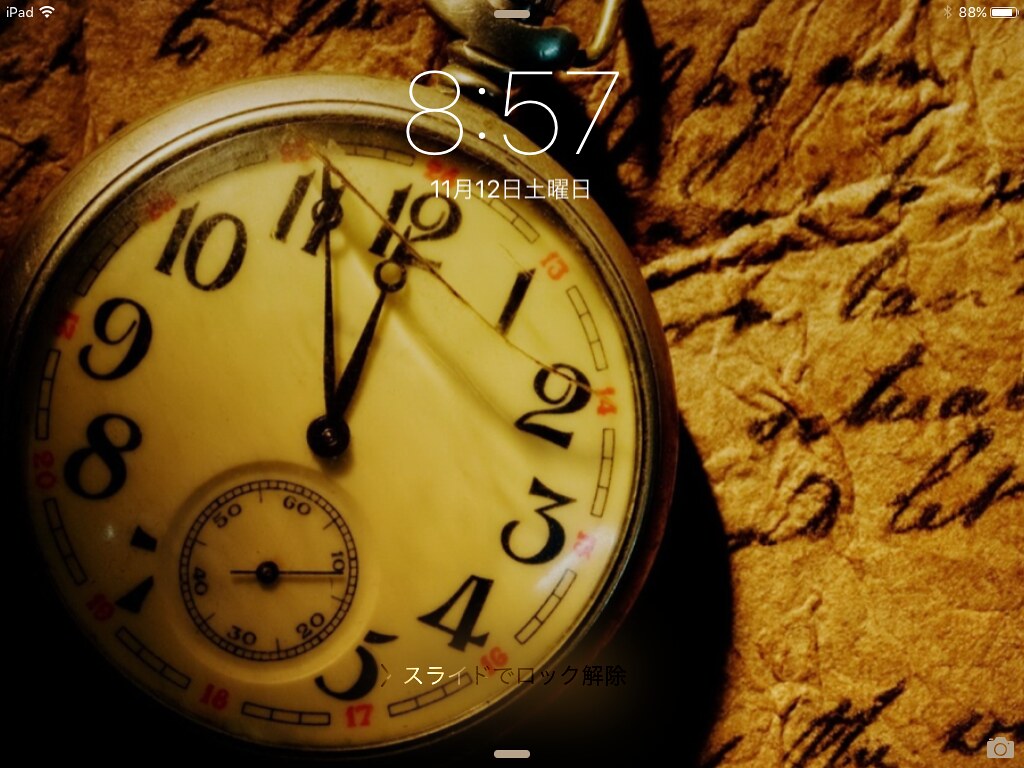The indoor color photograph prominently features a vintage brass or tarnished bronze pocket watch, positioned slightly left of center and mainly in the lower left quarter of the frame. The pocket watch face, displaying regular numerals from 1 to 12 along with an outer ring of military time, shows the time as 11:55 with its black hour and minute hands, and a smaller sub-dial for seconds where the hand points to 12 seconds. The watch crystal is notably cracked from the 11 o'clock to the 2 o'clock position. The watch is inclined to the right, causing the 12 o'clock marker to point diagonally. The background is a piece of parchment paper with elegant cursive writing in black ink, though the text is illegible. Overlaying this image are electronic device details: at the top center, digital text indicates "8:57," beneath which are the numbers "11," "12," and some Asian characters. The top left corner has the text "iPad" with a Wi-Fi symbol, while the top right shows "88%" alongside a battery icon. In the lower right corner, there is a silhouette of a photograph icon. Part of the pocket watch clip is visible but partially cut off at the top edge of the frame. The bottom left corner of the image fades into darkness.